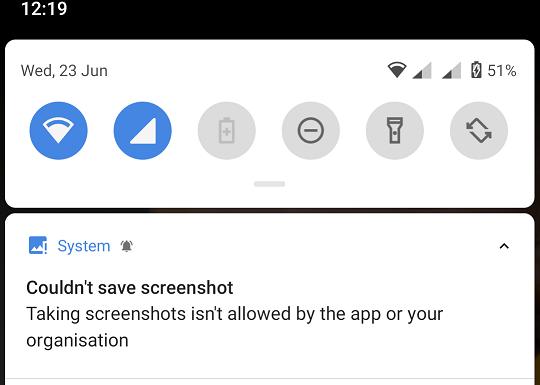The image is a zoomed-in screenshot from a cellphone display, revealing detailed elements of the device's status bar and notification area. The top portion of the screen is black, displaying "12:19" for the time. Positioned at the very top-left corner, the date "Wed, 23 June" is shown. Towards the right side of the screen, there are two triangle icons, representing a Wi-Fi connection, followed by a battery icon with a lightning strike inside it, indicating that the battery is at 51% and currently charging.

Below the status bar, there are six circular icons arranged in a row. The first two icons are blue: one resembles a Wi-Fi signal, while the other looks like a triangle. The remaining four gray icons include: a battery with a plus sign, a minus symbol inside a circle, a flashlight, and two arrows forming a loop. 

Toward the bottom of the screen, in blue text, it says "System" accompanied by an icon. Below this, in black text, it states, "Couldn't save screenshot. Taking screenshots isn't allowed by the app or your organization."